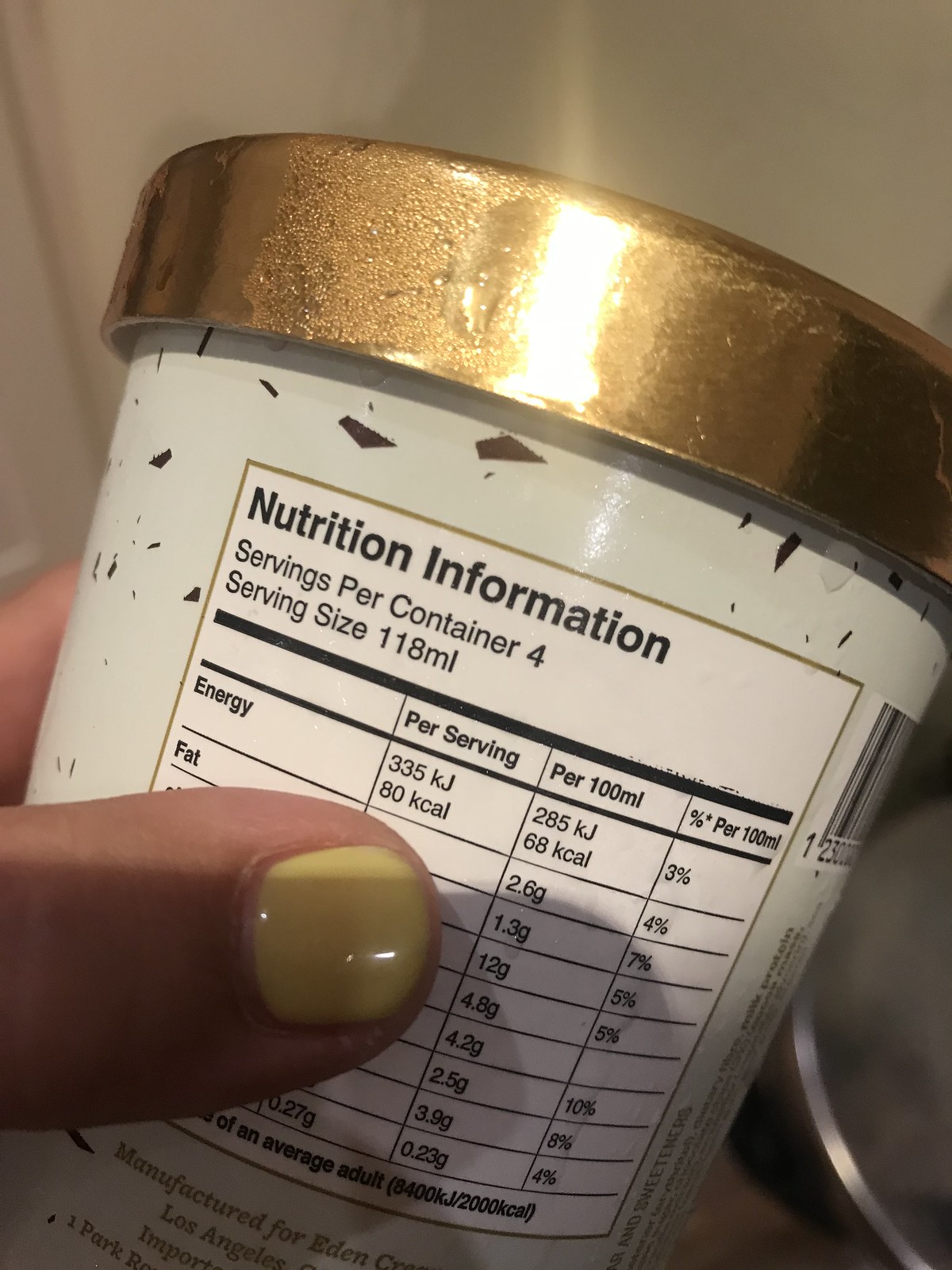This color close-up photograph, taken in a first-person POV style, features a small, white plastic container of ice cream, held in a person’s left hand. The person, likely female given her yellow-painted thumbnail, is capturing the image with their right hand. The container is adorned with floating and scattered small, four-sided dark brown chocolate pieces. The gold lid is tilted to the upper right and covered in moisture droplets, reflecting light and adding a sparkling effect.

We are looking at the back of the container, which prominently displays the nutrition information label. The label is primarily white with black text and bordered in gold. Key information includes that the servings per container are four, with each serving size being 118 milliliters. Energy provided is 335 kilojoules (80 calories) per serving. While the thumb covers part of the label, some nutritional details can be discerned, such as fat content at 2.6 grams per 100ml, equating to 4% of the daily value. Other nutritional values listed include 1.3 grams, 12 grams, 4.8 grams, 4.2 grams, 2.5 grams, 3.9 grams, and 0.23 grams per 100ml, with respective daily values of 7%, 5%, 5%, blank, 10%, 8%, and 4%. Shadows of the camera and hand are visible at the bottom quarter of the vertically aligned image.